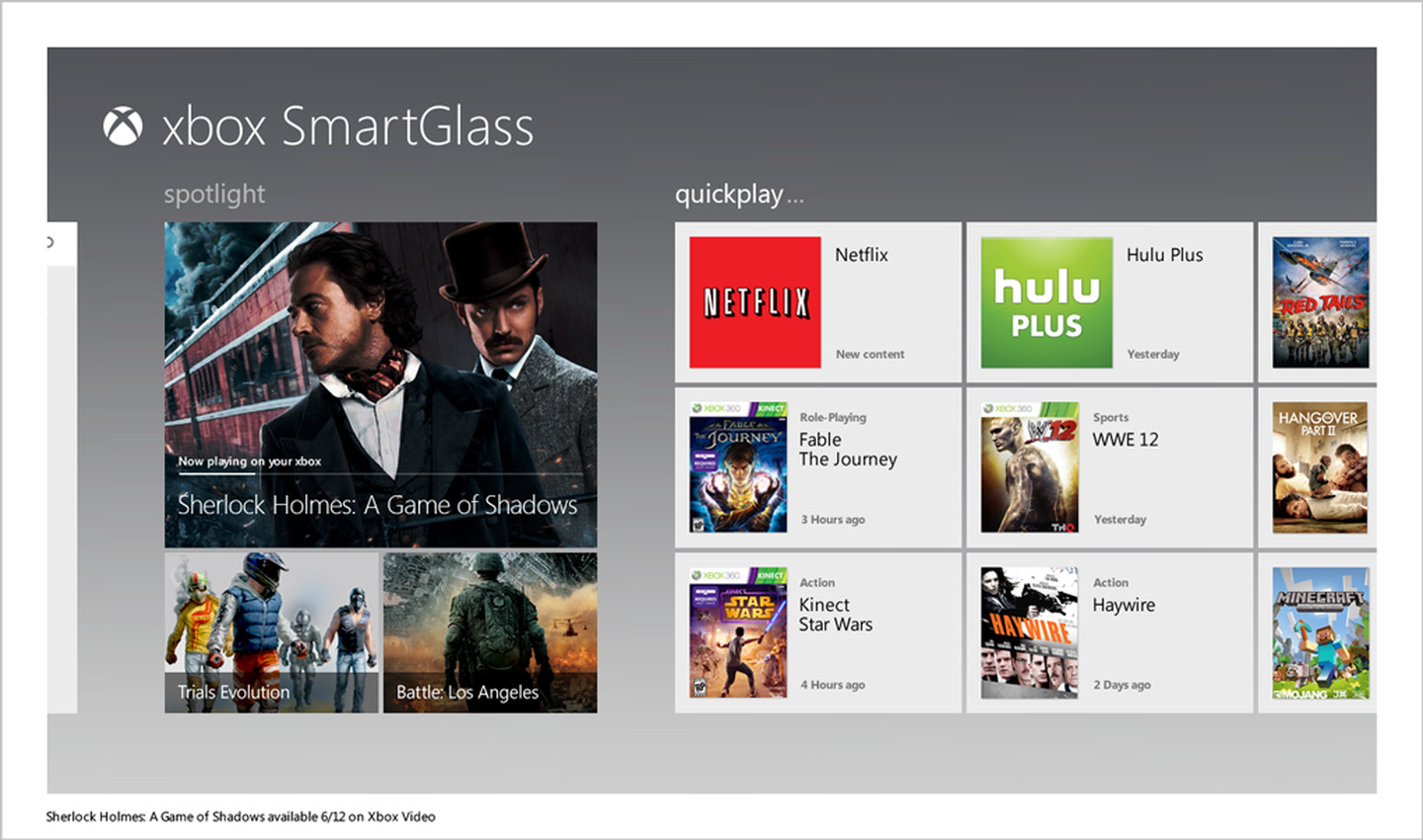A screenshot of the Xbox SmartGlass interface is shown. On the upper left-hand side, the words "Xbox SmartGlass" are displayed next to the Xbox logo. The interface is divided into two primary sections: the left section features a "Spotlight" area, while the right section is designated for "Quick Play."

In the "Spotlight" section on the left, there is a prominent thumbnail for "Sherlock Holmes: A Game of Shadows," indicating that it is "Now Playing on your Xbox." The thumbnail displays an image of two men standing in front of a train. Beneath this, there are two smaller thumbnails: one for "Trials Evolution" and another for "Battle Los Angeles."

The "Quick Play" section on the right showcases several highlighted apps and games. The first item is "Netflix," followed by "Hulu Plus." Next, there are thumbnails for "Fable: The Journey," "WWE '12," "Kinect Star Wars," and "Haywire."

Each element is neatly organized, providing users with an easy-to-navigate layout for accessing their favorite content on Xbox SmartGlass.